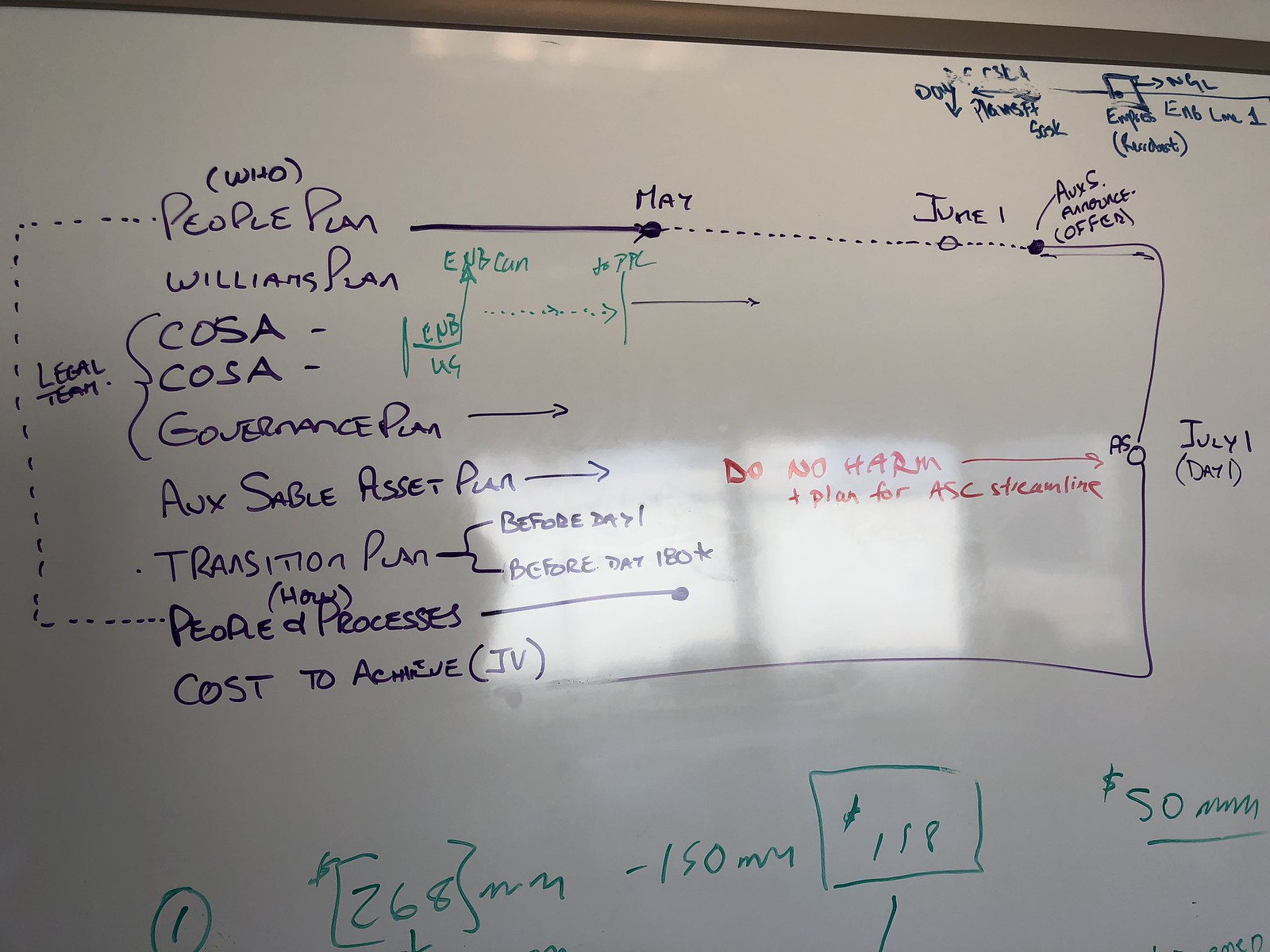The image showcases a whiteboard bordered in brown, filled with multicolored writing that outlines a project plan. On the left side, written in purple, are terms such as "who (people)," "people plan," "Williams plan," "COSA," "governance plan," "Aux Sable asset plan," "transition plan," "how," and "people and processes cost to achieve." The section also includes the words "legal team" and mentions of technical elements and legal aspects. In addition, a timeline is indicated across various colors (blue, green, red, and purple), with key dates such as "up to May," "June 1st," and "July day one." Further details include shorthand notes, budget numbers like "50 mm," "198," and other calculations written in green marker. The overall layout suggests a detailed project plan and timeline, with possible reflections of a window or a computer screen adding an extra layer of visual complexity.